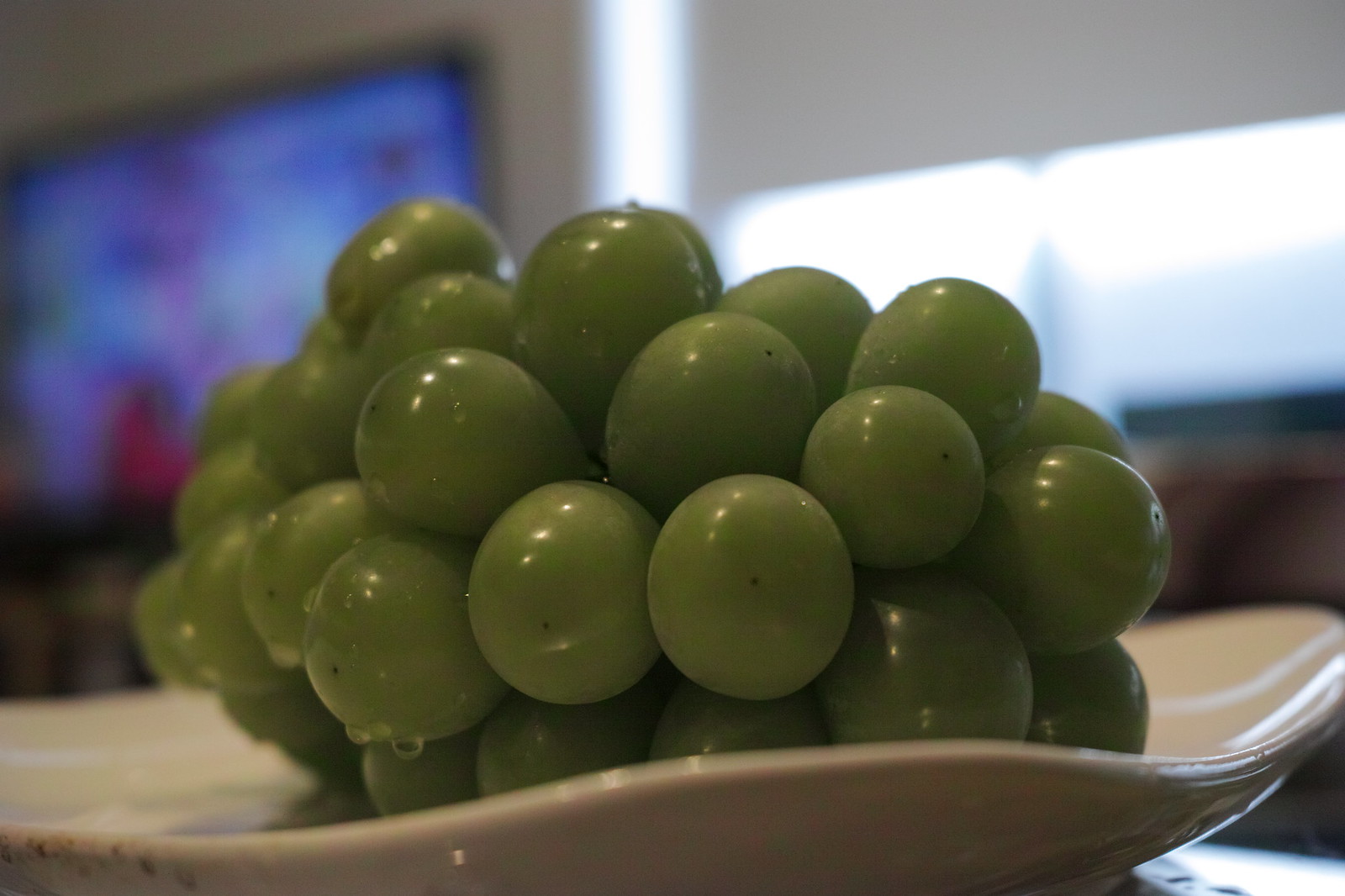This detailed colour photograph captures a close-up of a plate of round green grapes, freshly washed and glistening with water droplets. These grapes, each about two inches in diameter, are tightly clustered together in a bunch. Their light green hue and shiny surfaces, accentuated by small dots of reflected light, suggest freshness and readiness to be eaten. The grapes have a tiny black dot on the bottom, adding to their distinct appearance.

The grapes are arranged on a thick, white rectangular plate with wavy, curved edges. The background of the image is blurred, drawing focus to the vibrant grapes. In the upper left-hand corner, a blue, almost television-like screen is visible, showing the faint outline of a person wearing a red top. To the back right of the photo, light streams through a window, partially covered by blinds pulled halfway down, creating a bright area beneath. Below the window, a wooden surface is subtly visible. The scene overall exudes a casual yet detailed depiction of a moment at home, highlighting the grapes' fresh and inviting appearance.